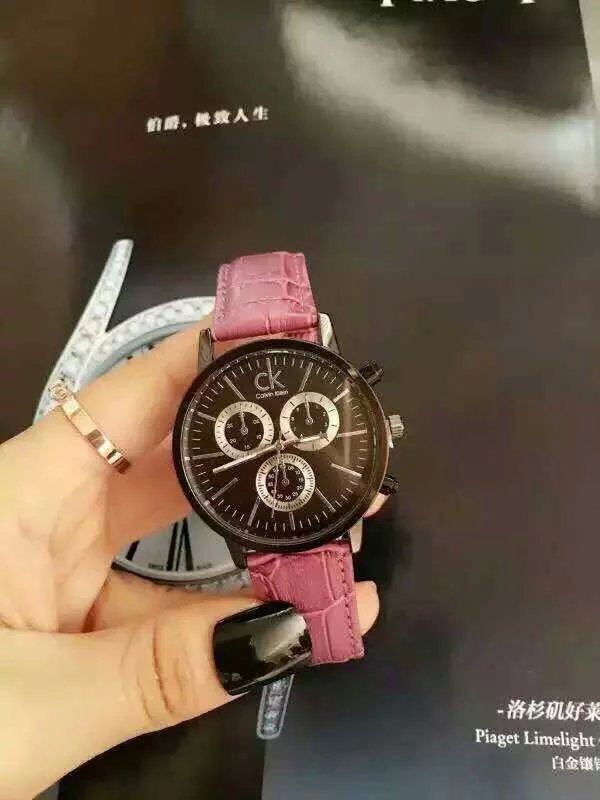A black tabletop serves as the backdrop for an elegant scene featuring a woman's hand adorned with black nail polish and a diamond ring with a gold band on her index finger. She is holding a sophisticated watch characterized by its pink leather strap, secured by metal bars at both ends. The watch face is a deep black, marked by sleek silver minute, hour, and second hands. Notably, the watch also features three additional sub-dials, though their specific functions are unclear. The branding "CK Calvin Klein" is prominently displayed at the top of the watch face, accompanied by "Kayaget Limelight" in the bottom right corner, flanked by Chinese and Japanese text. In the background, a clock face bordered with what appears to be diamonds adds an extra touch of luxury. Additionally, there are Chinese or Japanese characters situated towards the upper center of the image, contributing to the overall exotic and luxurious ambiance.